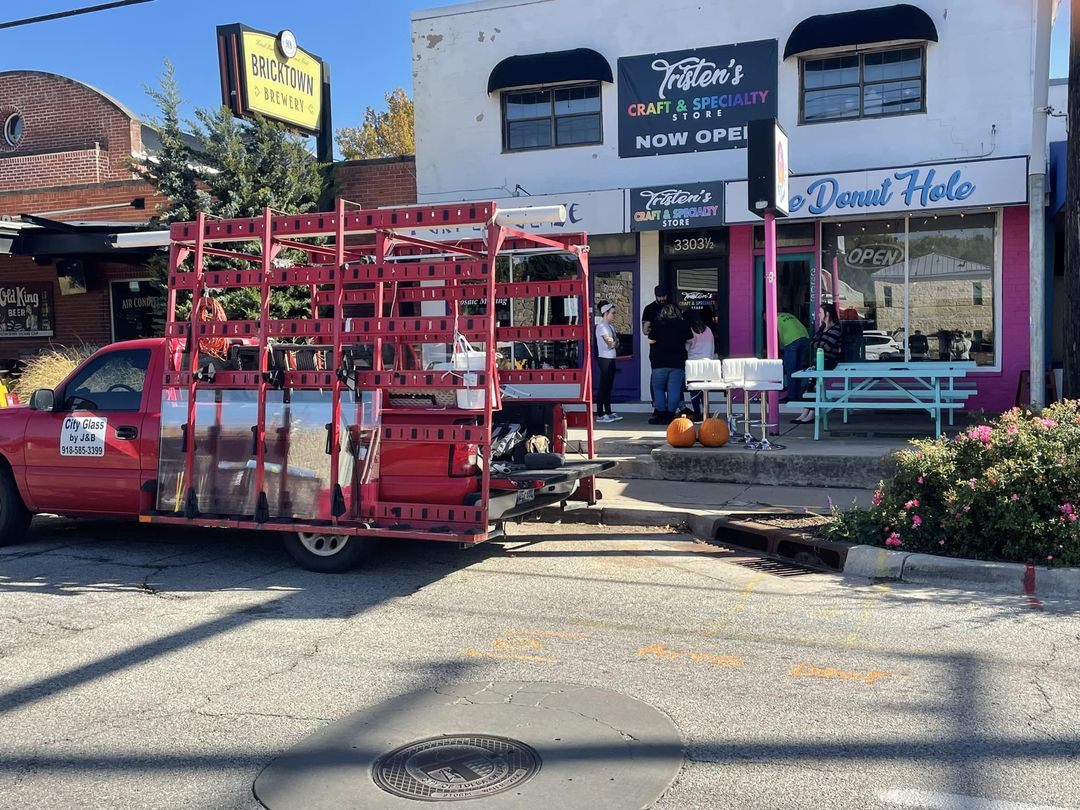The photograph captures a lively daytime street scene in a small downtown area. Dominating the composition is a large red work truck parked on the left side of the street, adorned with a metal rack likely used for transporting glass or mirrors. The door of the truck features a slightly obscured white square sign with black text that reads "City Glass by J&B" along with a phone number. Above, the sky is a clear, uninterrupted blue. Adjacent to the truck and partially blocking part of the view is a storefront for "Tristan’s Craft and Specialty Store Now Open," which boasts a sign with "Tristan's" in white cursive, "Craft and Specialty" in rainbow colors, and "Store Now Open" in white text. In front of this store, a man in a black shirt engages in conversation with two people in white shirts and another individual in a neon green safety shirt can be seen near the adjacent "The Donut Hole" storefront. This neighboring shop is labeled with blue cursive text and has a blue picnic table outside its window, which reflects the vibrant street scene. Additional details include a manhole cover on the asphalt street, some curbside landscaping, and two pumpkins placed near the storefront, enhancing the quaint, communal atmosphere of the setting. To the left, though obscured by the truck, is a brick building with a sign indicating "Bricktown Brewery."